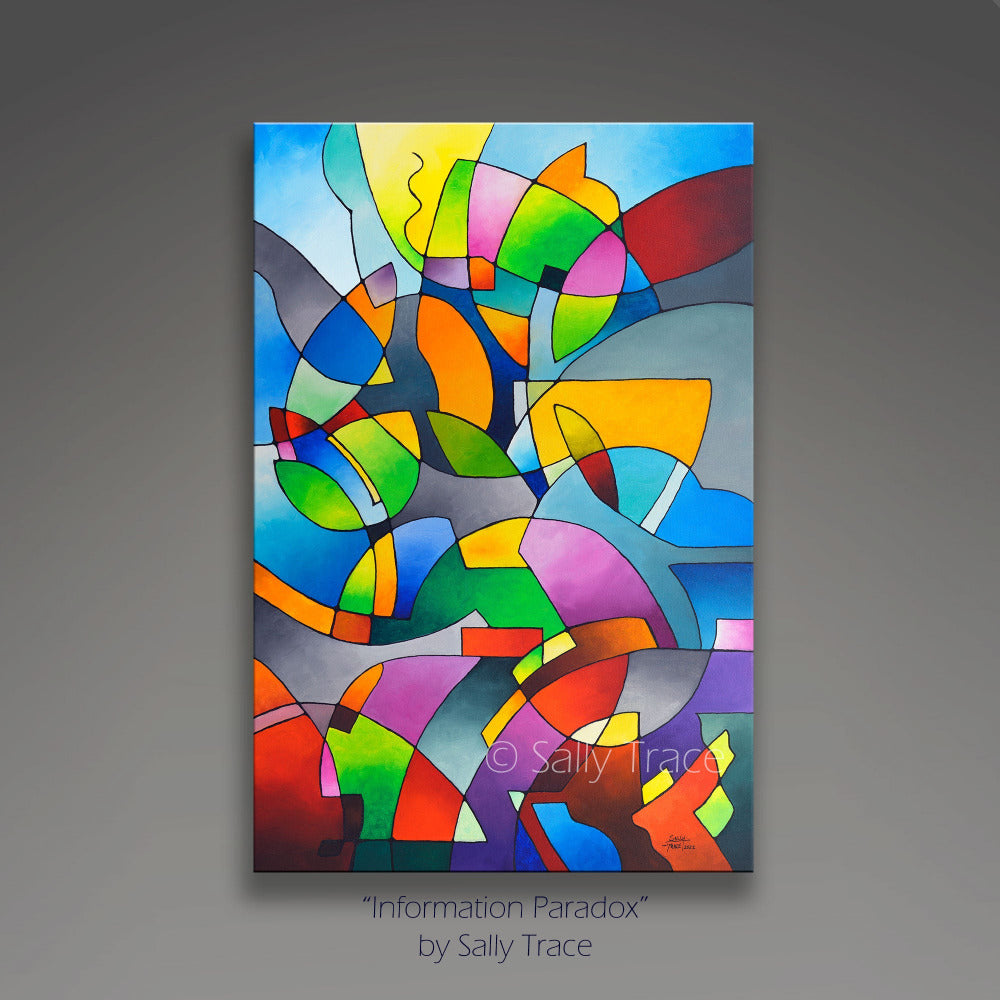This is a professional image of a large art print on canvas, presented against a gray background to give the impression of being hung on a wall, complete with a slight drop shadow. The painting, titled "Information Paradox" by Sally Trace, features a vibrant Picasso-style composition filled with various geometrical shapes such as triangles, circles, ovals, and more, all outlined in black. The colorful mosaic includes an array of hues including yellow, red, pink, blue, green, orange, purple, magenta, and more, seemingly arranged in a random yet visually striking manner that resembles postmodern stained glass. A white watermark reading "© Sally Trace" is prominently displayed over the canvas, and the artist's signature can be found at the bottom. Below the painting, there is centered text that reads "Information Paradox by Sally Trace."